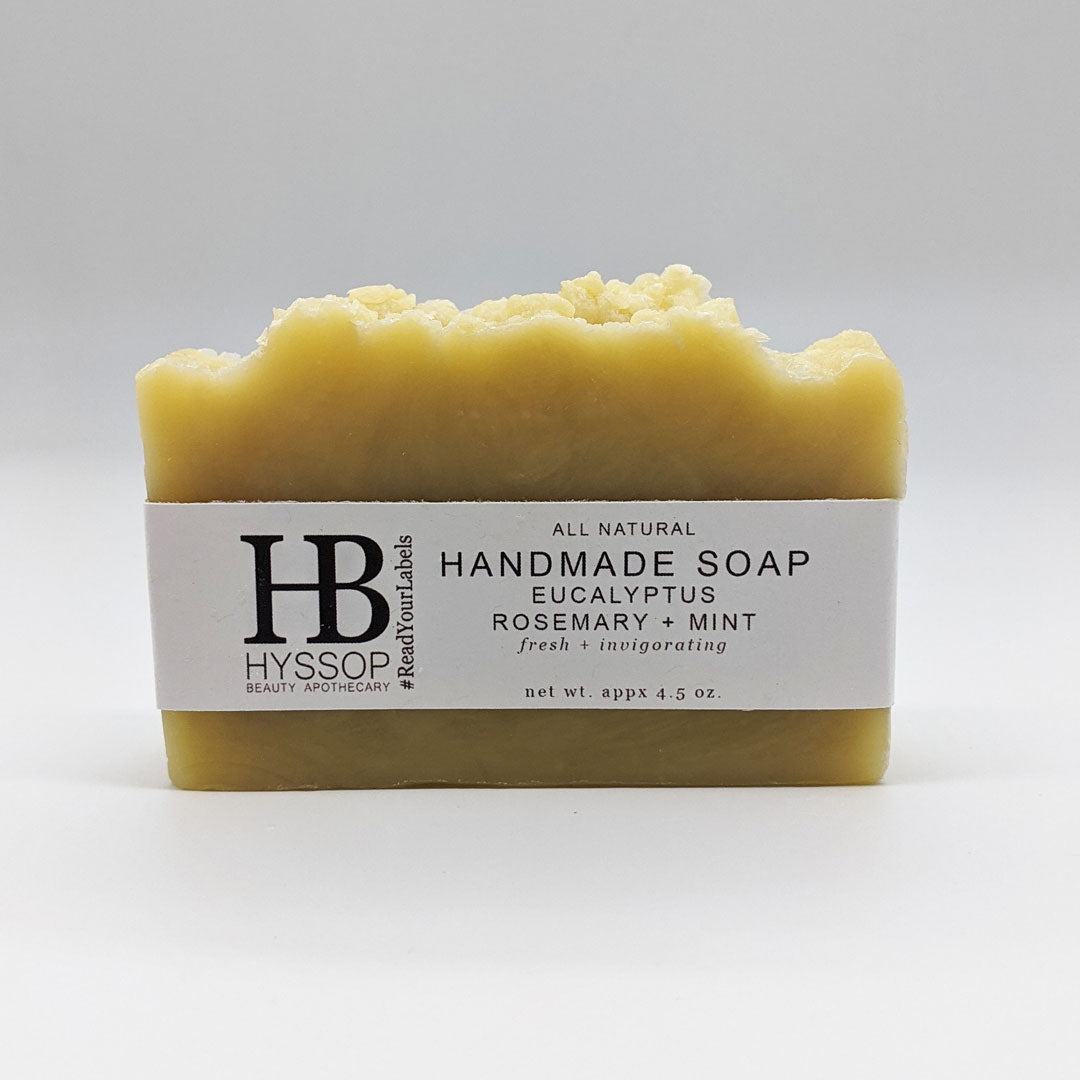The image features a vividly yellow, handmade bar of soap with a somewhat irregular, rugged top and smooth, rectangular sides. The soap is wrapped in a cardboard label that prominently displays the brand name "Hyssop Beauty Apothecary" along with the initials "HB." The label includes a hashtag reading "#ReadYourLabels" along one side, all in black font. It also highlights that the soap is "All Natural Handmade Soap" in eucalyptus, rosemary, and mint scents, described as "Fresh & Invigorating" in cursive text. The net weight is listed as approximately 4.5 ounces in smaller print. The entire setup is set against a clean, completely white background.